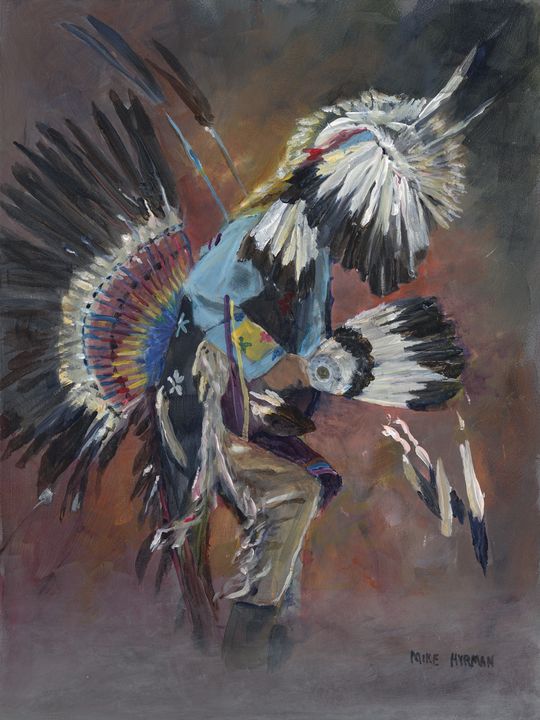This vertical rectangular image, either a photograph or a detailed artist's drawing, portrays an intricate scene from an American Indian ceremony. The focal point is a Native American man captured mid-dance, seen from the side. He is adorned in khaki-colored buckskin pants and a blue shirt with feathers. His attire features elaborate feathered and furry headgear that completely covers his head from the side. A large fan-shaped array of feathers extends from his back, creating a striking visual effect. In his hand, he holds a feathered device from which some feathers appear to be falling. The background of the image is a rich brownish-gray with red and orange tones, adding depth and warmth to the scene. At the bottom right corner, the artist's signature, "Mike Hyrman," is clearly visible in black text.